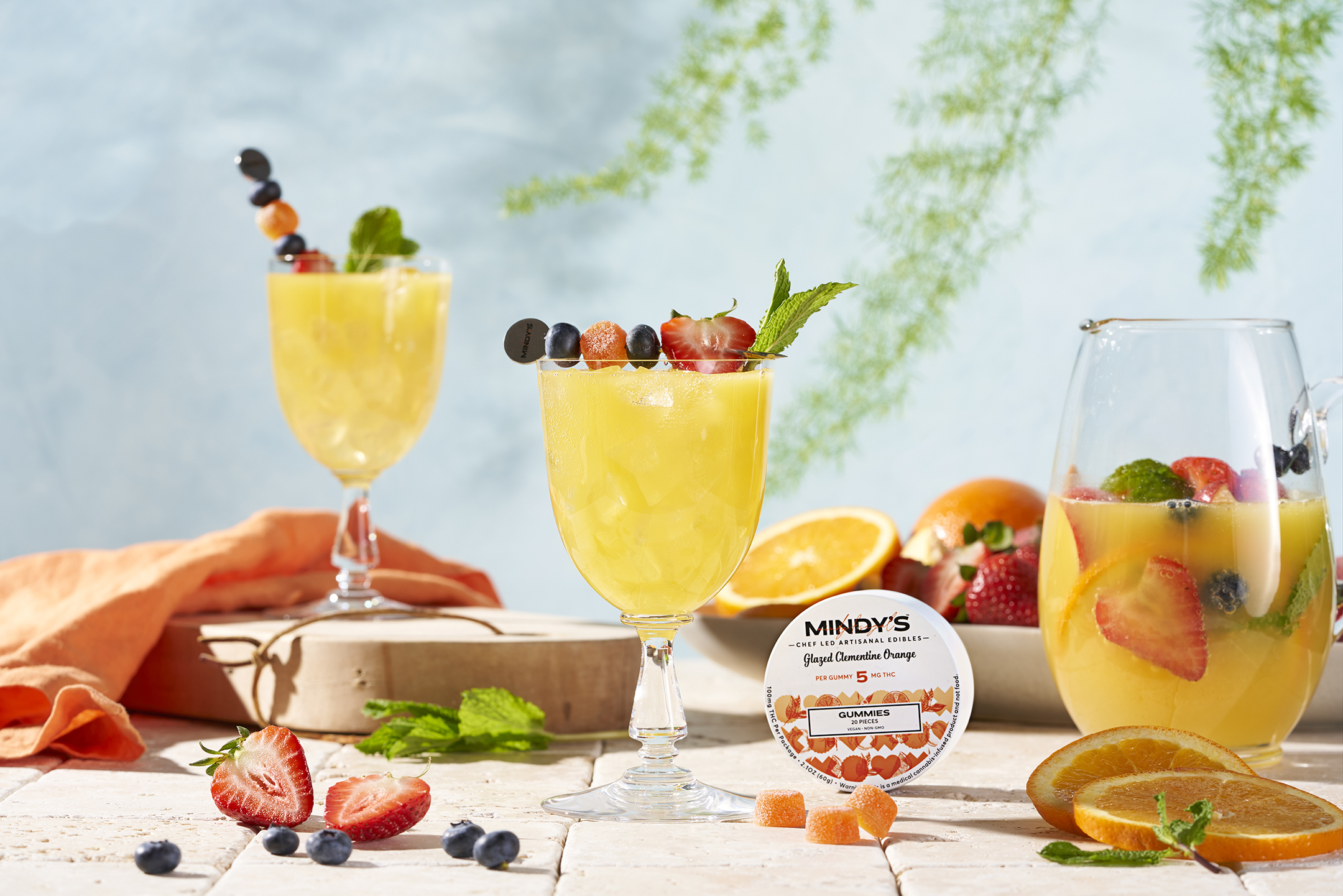This professional food photograph captures a beautifully styled table scene set against a backdrop of a cloudy, blue-gray sky with green tree fronds hanging in from the upper right. Central to the image are three beverages, each showcasing a vibrant yellow-orange liquid, presumably a type of iced juice. The leftmost drink, raised on a wooden block, is presented in an elegant goblet and adorned with a skewer holding blueberries, strawberries, and mint leaves. The middle drink, also in a goblet, mirrors the left one but has the skewer lying horizontally across the top. 

To the right, a rounded glass shows a half-filled drink with fruit pieces, likely including strawberries, orange slices, and mint leaves. The beverages sit on a light-beige, speckled tile surface, which may be part of an outdoor table. Scattered around are fresh fruits—sliced strawberries, blueberries, and orange segments.

Prominently featured at the center bottom is a circular tin labeled "Mindy's" advertising "Glazed Clementine Orange Gummies," with a few gummies placed outside the container. Adding to the arrangement is an orange kitchen towel in the bottom left, adding a pop of color to the scene.

This meticulously arranged setting offers a refreshing and inviting display, emphasizing the vibrant colors and textures of both the drinks and accompanying fruits.